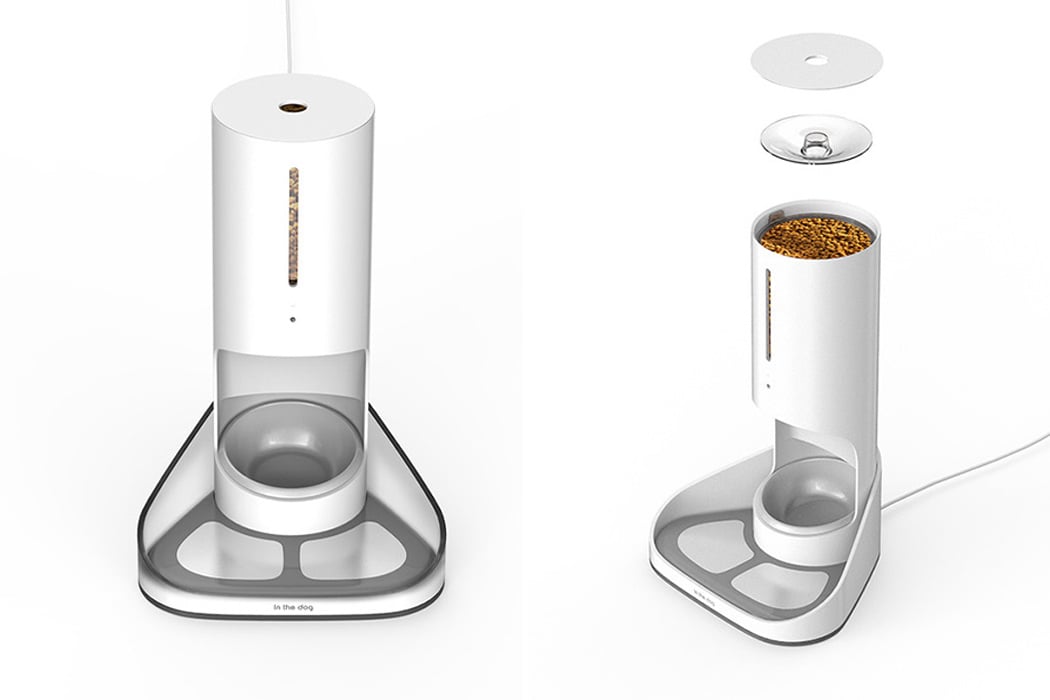The image depicts an automatic dry food feeder designed for pets, displaying both a frontal and a side view against a slightly off-white background. The feeder features a long white cylinder with a vertical window in the middle to monitor the food level. This cylinder is mounted on a triangular base that includes a centrally placed bowl where the food is dispensed when automated. 

From the frontal view on the left, we can see the window showing the filled food level, and the base with the triangular bowl arrangement where the food is delivered. The side view on the right reveals additional details: a power cord extends from the back to power the device, and there's a detailed look at the cylinder, which has a cover and an additional plastic piece on top. The top section of the feeder is shown partially open with its dual-layered seals lifted, illustrating where the dry food is loaded. The base also features a design that can potentially allow the bowls to be positioned either to the left or the right, accommodating multiple pets. The device is primarily white and seems to have some writing at the bottom, possibly related to its function as a pet feeder.